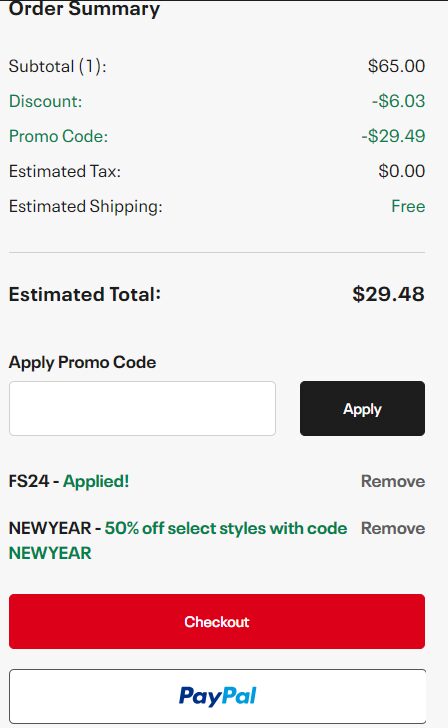**Detailed Caption:**

This is a detailed screenshot captured from a smartphone, showcasing the final order summary page following a completed purchase. At the top left corner, the heading "Order Summary" is prominently displayed. Below this heading, the breakdown of the order is listed.

The first item in the summary is the "Subtotal" with an adjacent marking of "1," indicating a single item in the order. The subtotal amount is $65. Following this, a "Discount" of $6.03 has been applied. A promotional code has further reduced the price by $29.49, noted as "-$29.49."

The tax for the order is estimated at $0, and shipping is indicated to be free. As a result of these deductions, the "Estimated Total" is bolded and shows an amount of $29.48.

Directly below this total, there is a section where an additional promotional code can be applied. The text "Apply Promo Code" is positioned above a text field, next to a black button labeled "Apply." 

Beneath this section, the successfully applied code "FS-24" is highlighted with the word "Applied" in green text. The promotion "NEW YEAR" is also visible, with an accompanying note that states "50% off selected styles with code NEWYEAR," also written in green text.

At the very bottom of the page, a large red button labeled "Checkout" is prominently displayed. Below the checkout button, an alternative option to pay with PayPal is provided with a corresponding button.